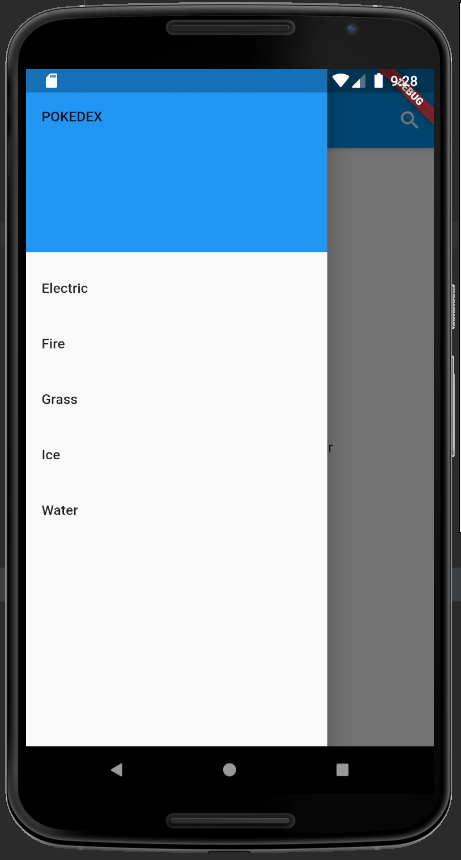In this image, we observe a mobile device with various interface elements. At the top right corner, the screen displays the current time, 9:28, alongside the battery bar indicator and the Wi-Fi signal indicator. On the top left, there is an icon representing storage status. The menu page prominently features text options including "Poké-e," "Pokédex," "Electric," "Fire," "Grass," "Ice," and "Water," each set against a background palette of white, blue, and black. Additionally, the mobile device is equipped with two speakers, with one positioned at the top and the other at the bottom, enhancing its audio output capabilities.